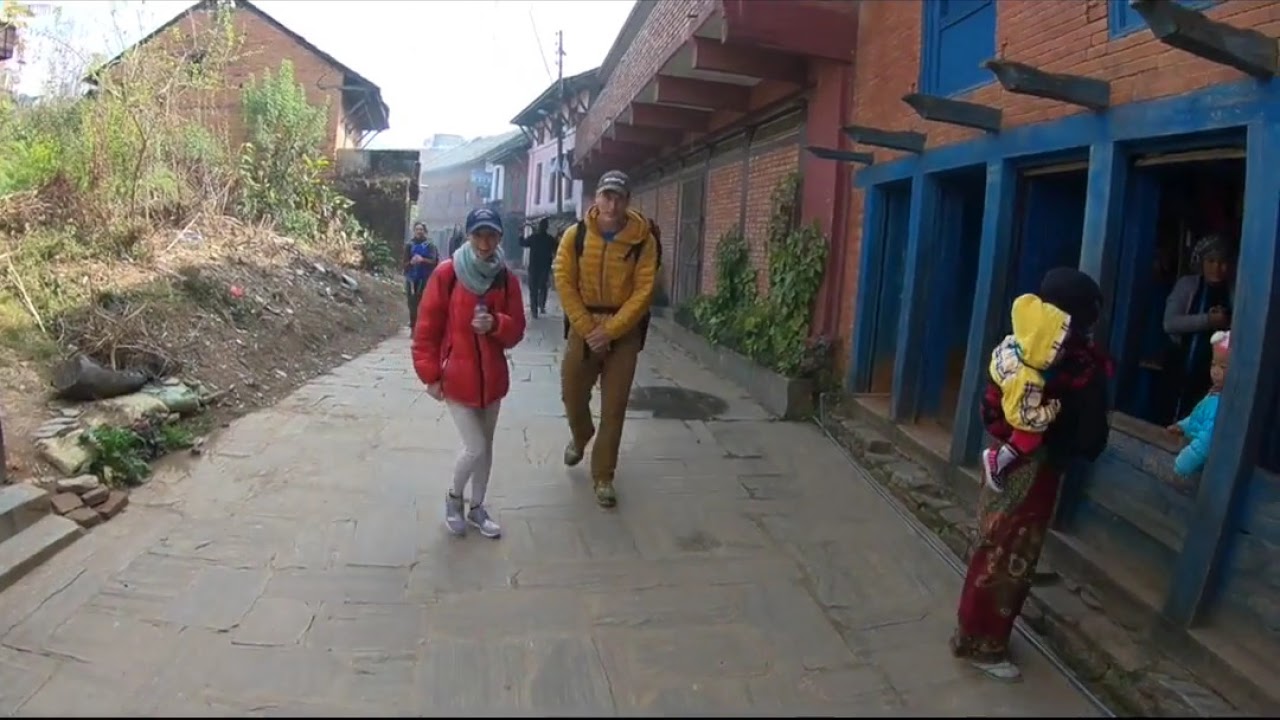In the photo, a couple walks along a stone-paved walkway through a rural village. The woman, centered in the image, wears a red jacket, blue scarf, blue baseball cap, and white pants with gray shoes. To her right, the man wears a mustard-colored puffer jacket, gray cap with white writing, tan pants, and gray shoes, carrying a black-strapped backpack. The walkway is flanked by brick row houses on the right, with the nearest building sporting blue window and door frames. On the left side, a small slope is covered in brown vegetation and scattered trash. Additional villagers, including children and an adult holding a child, can be seen further along the pathway and near the houses, evoking the sense of a close-knit, vibrant community.